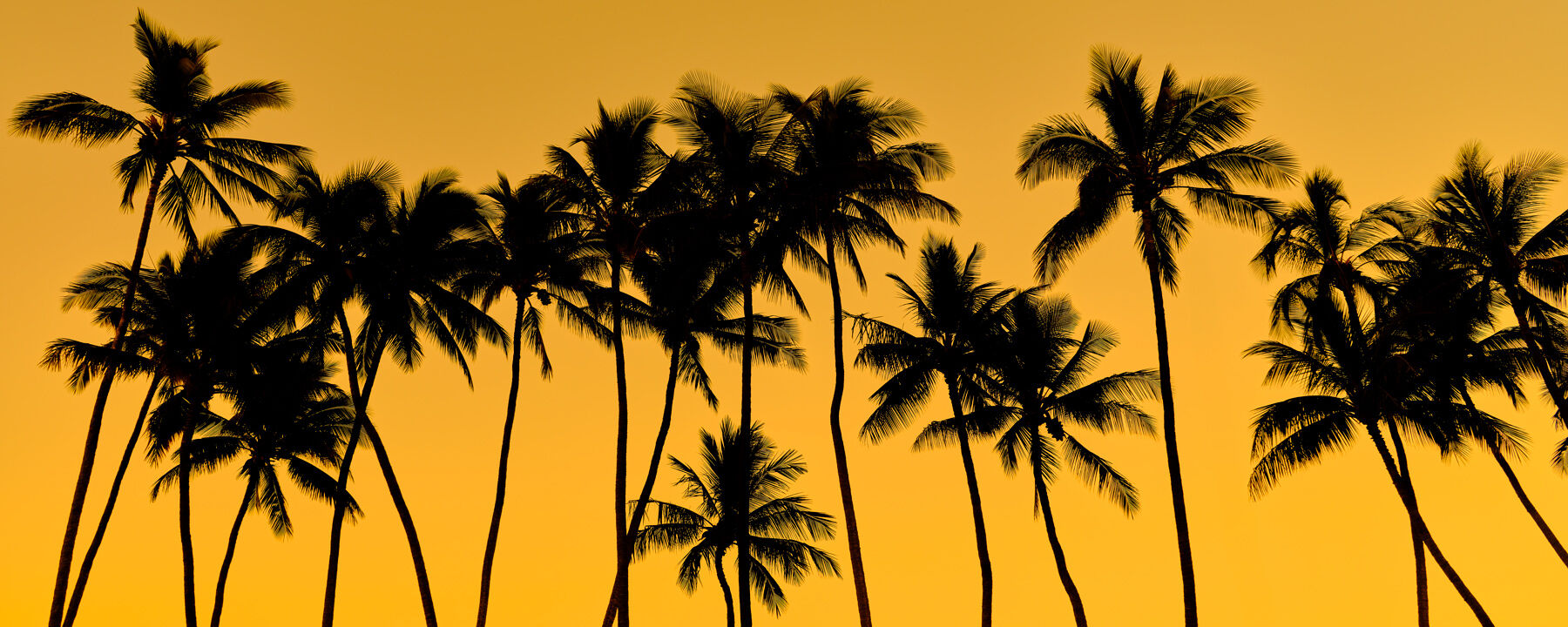This is a horizontal image of around 15 to 20 tall, skinny palm trees, depicted as dark silhouettes against a rich yellow-orange background, suggesting it was taken around sunrise or sunset. The image is likely AI-generated but boasts exceptional detail, particularly in the trunks and the fronds of the palm trees. The trees appear humongous, with heights that could be estimated between 30 to 40 feet, and they are spaced closely together, creating a dense cluster. Although the green of the palm leaves is not visible due to the silhouette effect, the dark black color of the palms contrasts strikingly with the background, enhancing the visibility of each individual frond. The backdrop of the image, a darker, non-neon yellow, provides a beautiful contrasting canvas that highlights the intricate details of the palm tree silhouettes. This scene evokes a beach theme, despite there being no direct indication of the geographical location. The perspective of the image makes it seem as though the viewer is looking up and out at the towering palms from ground level.